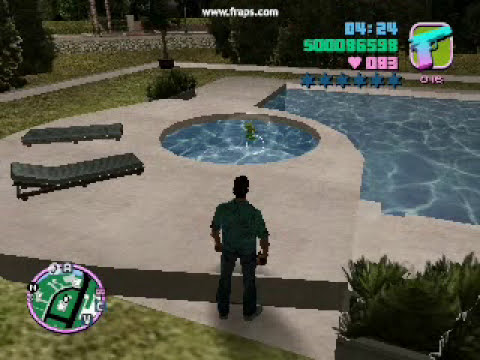The image is a grainy, computer-generated screen capture from a video game, likely from the GTA series. At the top of the screen, a website URL, "www.fraps.com," is displayed in white letters, though it is somewhat blurry to read. The upper right-hand corner of the screen shows game stats including a score, a counter, and an icon of a gun in teal and lavender colors, as well as a timer at 4 minutes, 24 seconds, and an 83 next to a pink heart icon, hinting at the player's health or life status. In the scene, a man, presumably the player's character, is standing in front of a uniquely shaped pool that has a curved corner section containing a circular pool, likely a hot tub. The pool area is surrounded by greenery with shrubs and trees, and there's a stone wall in the background. To the left are two lounge chairs positioned beside the circular hot tub section. The water in both pools reflects light and shows faint rippling lines. The entire setup suggests a backyard setting during daytime.